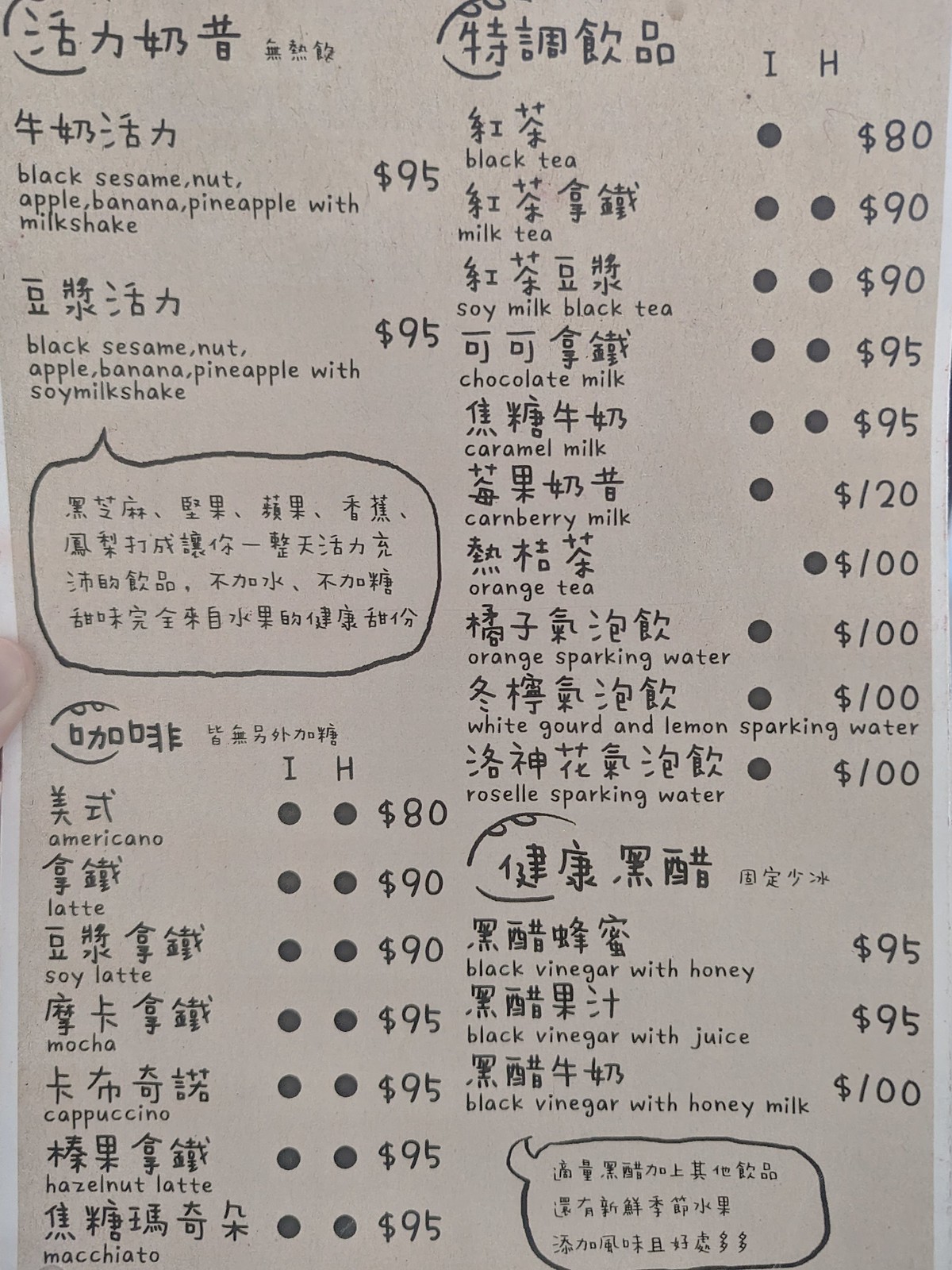The image depicts a bilingual menu printed on medium grey paper with black ink, showcasing both Japanese characters and English text. It features a variety of beverages, each with distinct pricing and annotations. The menu is divided into sections, with a mixture of drinks including milkshakes, coffees, teas, and sparkling waters.

In the milkshake section, notable items include:
- Black Sesame Nut, Apple, Banana, and Pineapple Milkshake priced at $95.
- A similar combination with soy milk called Black Sesame Nut, Apple, Banana, and Pineapple Soy Milkshake.

The coffee section in the lower left corner lists:
- Americano at $80.
- Latte, Soy Latte, Mocha, and Cappuccino each at $90 or $95.
- Hazelnut and Macchiato, both priced at $95.

On the right side, the tea and milk section includes:
- Black Tea for $80.
- Milk Tea and Soy Black Milk Tea both at $90.
- Various flavored milks such as Chocolate Milk, Caramel Milk, and Cranberry Milk, with prices ranging from $95 to $120.

Sparkling water options include:
- Orange Tea, Orange Sparkling Water, White Gourd and Lemon Sparkling Water, and Roselle Sparkling Water, each priced at $100.
- Unique beverages like Black Vinegar with Honey, Black Vinegar with Juice, and Black Vinegar with Honey Milk, ranging from $95 to $100.

Annotations on the menu feature columns labeled "I" and "H," accompanied by black dots next to the prices. Some items have dots for both "I" and "H," while others have dots for only one or none. This notation system appears to indicate specific attributes or categories for the drinks, though the exact meaning remains unclear.

Additionally, the menu contains playful elements such as speech bubbles resembling those found in comic books, adding a whimsical touch to the visual presentation.